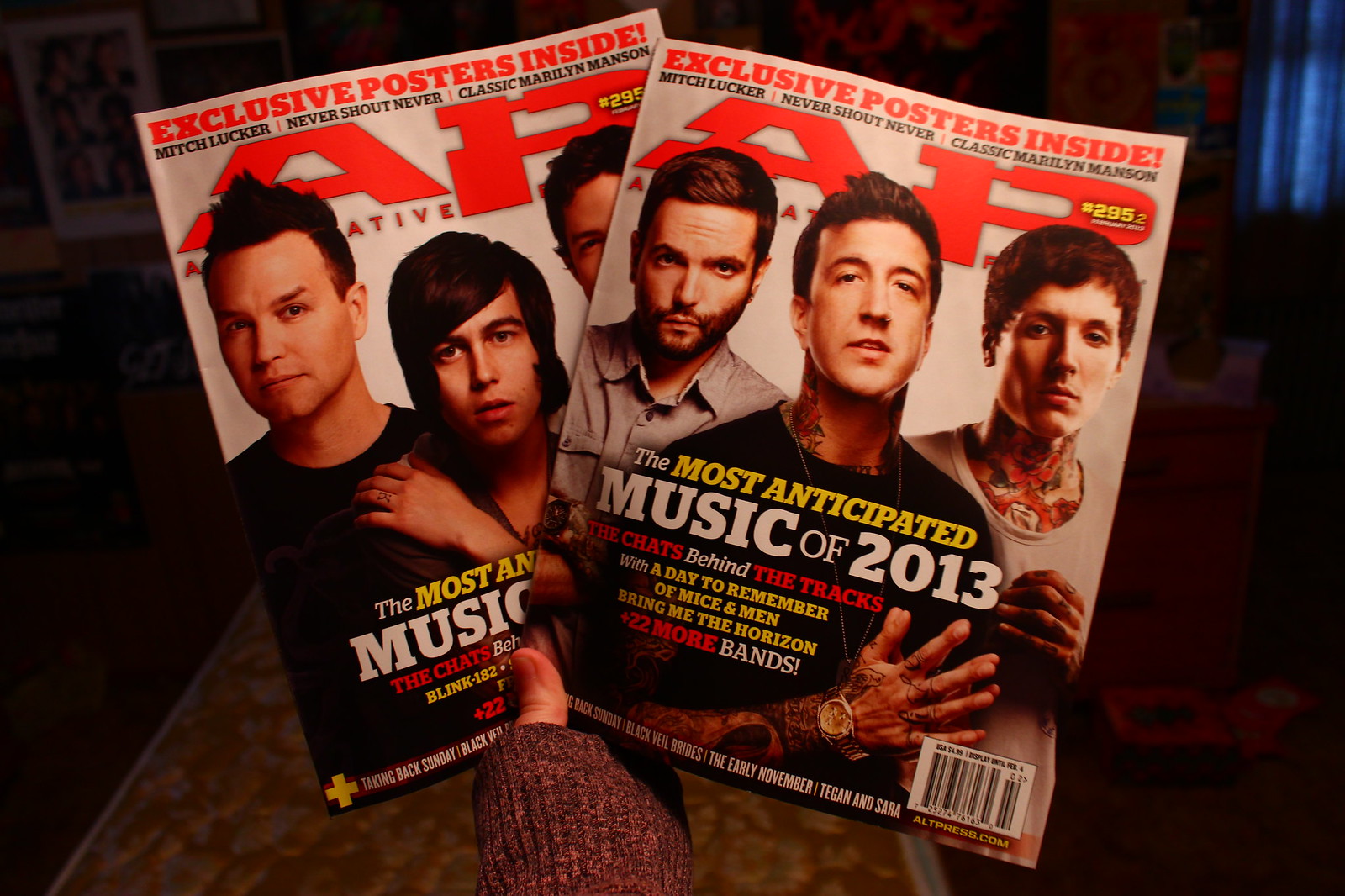In this vibrant and detailed image, we see a person, wearing a darkish pink sweater with their thumbs sticking out, holding up two almost identical alternate covers of an issue of Alternative Press magazine. Each cover prominently features three musicians with dark hair, but they belong to different bands. The magazine in the foreground (on the right) displays the headline, "The Most Anticipated Music of 2013," along with the magazine's large "AP" logo and top text that reads, "Exclusive Posters Inside: Mitch Lucker, Never Shout Never, Classic Marilyn Manson," and mentions bands like A Day to Remember, Of Mice & Men, and Bring Me the Horizon, plus 22 more bands. The left cover, although partially cut off, displays similar key text about "The Most Anticipated Music" and features members from the band Blink-182. The scene is set in what appears to be a bedroom, with a rug on the floor, and a dresser or nightstand with drawers behind the magazines, along with a box visible on the floor, adding to the lived-in feel of the space.